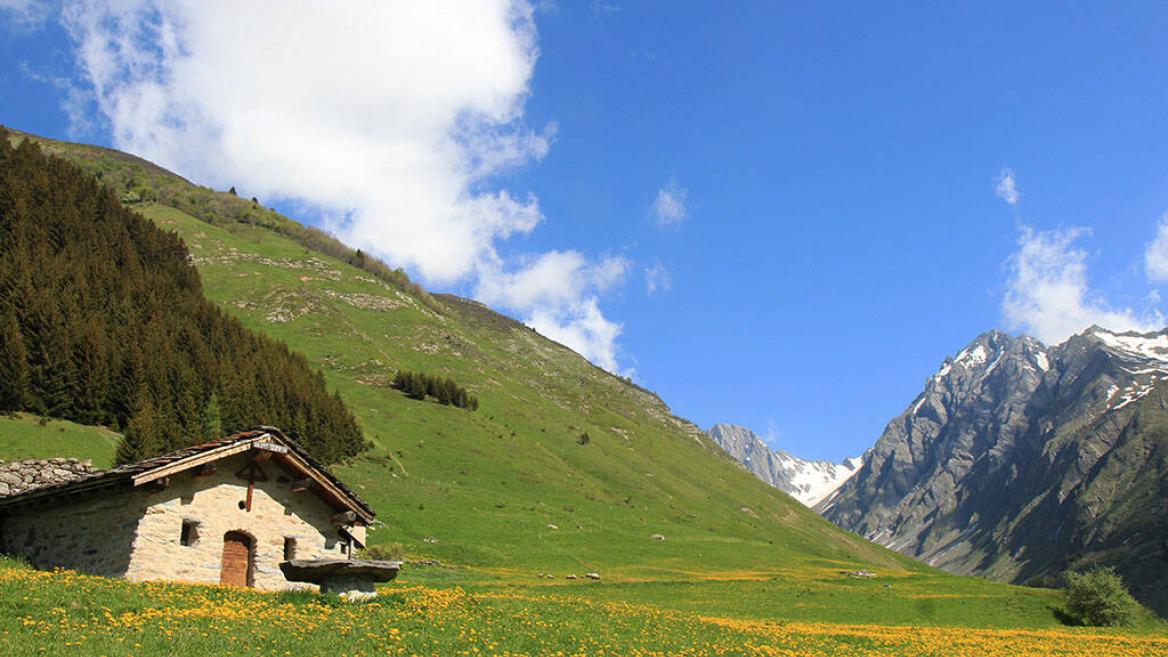This photograph captures a breathtaking outdoor scene on what appears to be a spring day. The sky is a brilliant blue with scattered puffy white clouds, creating a serene backdrop for the landscape. On the right side of the frame, a craggy, gray mountain range rises with patches of white snow clinging to its peaks. To the left, a verdant hill rolls gently upward, dotted with lush green grass and pine trees, suggesting the terrain ascends into another mountainous area.

In the foreground, a quaint stone cottage with an off-white façade sits on the bottom left. This old yet well-maintained structure features a reddish-brown, wooden arched doorway and two small windows, one on each side. The cottage has a peaked, brown-tiled roof, which adds to its rustic charm. In front of the cottage stands a small stone structure that appears to function as either an old fountain or possibly a table, though no chairs accompany it. Further enhancing the picturesque scenery, the foreground is adorned with tall grass and blooming yellow wildflowers, their color contributing to the springtime atmosphere. A couple of animals, likely cows or sheep, can be seen grazing in the distance, adding life to this idyllic mountain valley. Scattered rocks and a small stone wall complete the pastoral scene.